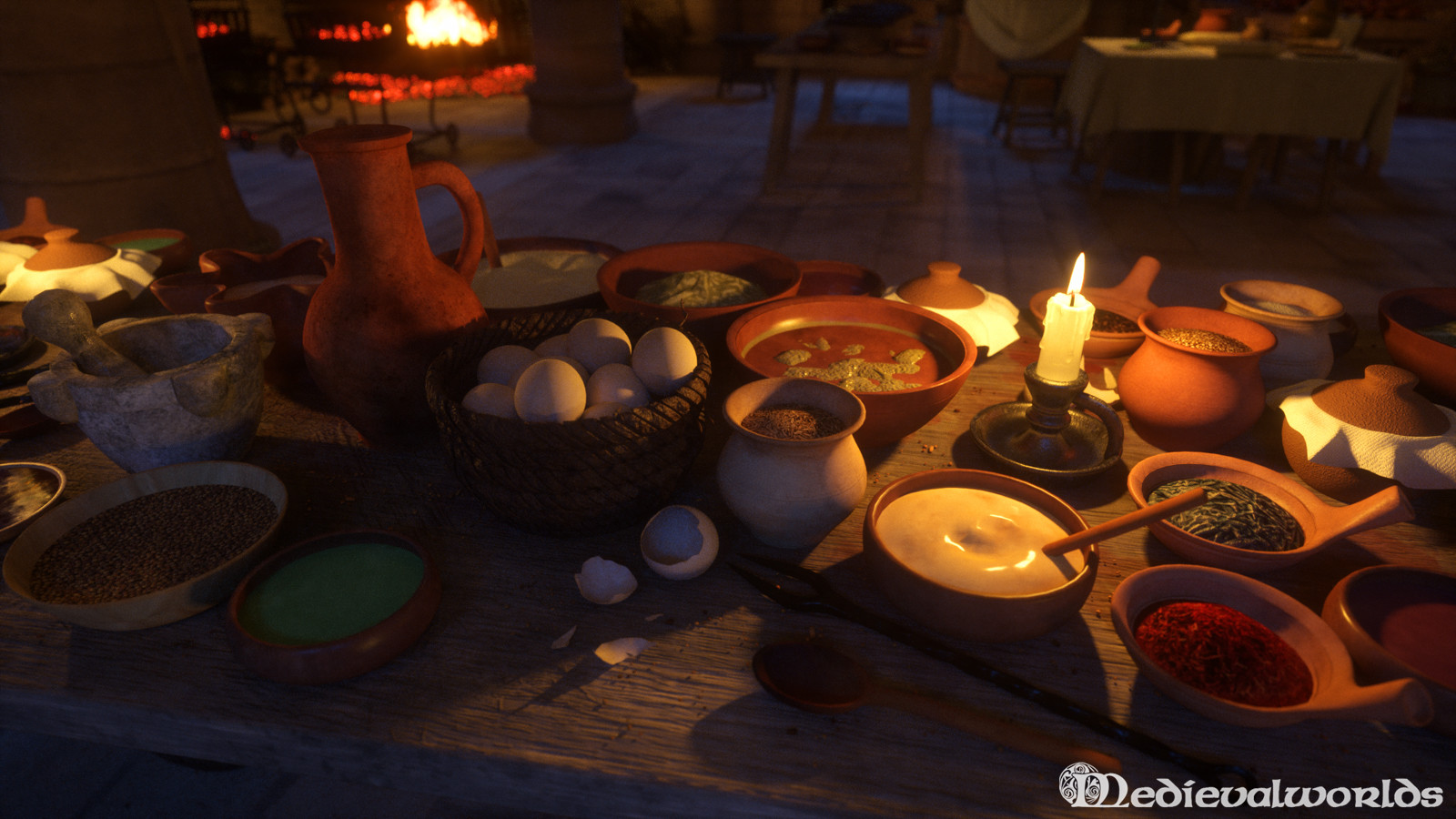In this AI-generated digital image, a dimly lit medieval kitchen table is showcased, illuminated predominantly by candlelight and the warm glow from a distant fireplace. The old wooden table is laden with an array of food items and various kitchen implements. Central to the scene is a wicker basket filled with white eggs, accompanied by a gray-black stone mortar and pestle for grinding herbs. Surrounding these are numerous earthenware and clay bowls of different shades, some containing dried red and green spices, a creamy liquid that may be soup or stew, and an assortment of rustic wooden bowls and spoons. A striking element is a silver metal candle holder with a white candle providing a soft light to the tableau. Additionally, there are props such as a rustic metal pitcher, likely for water, and a white bowl of sauce. The setting extends to a stone-tiled floor, brown stone block columns, and wooden tables and chairs, evoking the ambiance of a medieval tavern. A line of text reading "Medieval Worlds" is prominently displayed at the bottom right-hand corner, reinforcing the historical theme of the image.